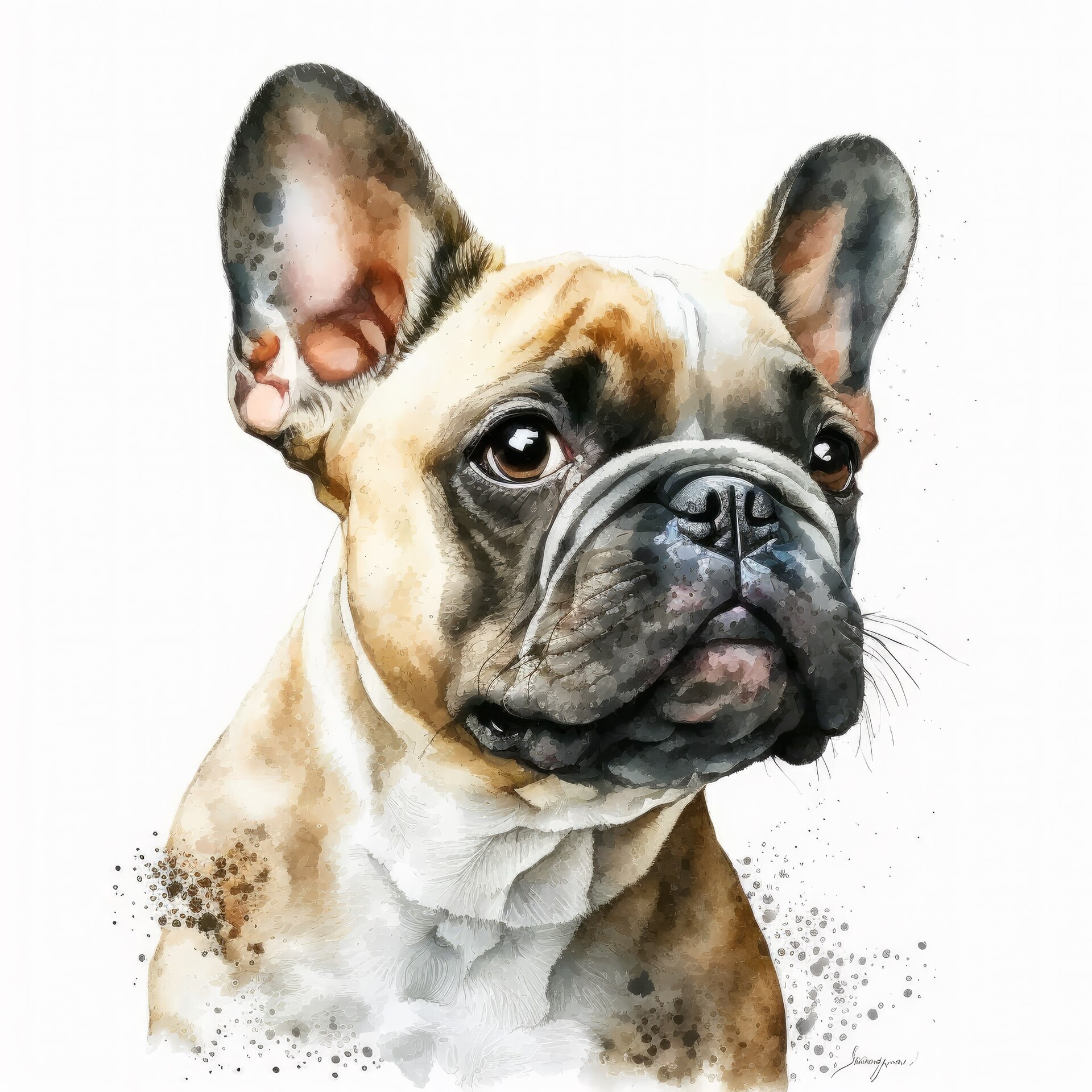This painting depicts a French Bulldog in a front-facing profile against a white background. The dog has a prominent, wrinkled face with dark, expressive brown eyes outlined with black. The top of its head features a distinctive white line that extends down towards its snout, which has black and splotches of cyan and green near the mouth area, ending in slight pink speckles. The dog's fur is a mix of tan, brown, and white, with a white patch covering its chest and extending from its chin down to the point where its lower body is cut off. The ears are erect and attentive, with pink interiors and dark black outer edges. Surrounding the dog are speckles of brown and gray paint, giving an impression of mud splashes. The artwork also bears a difficult-to-read signature at the bottom right corner.